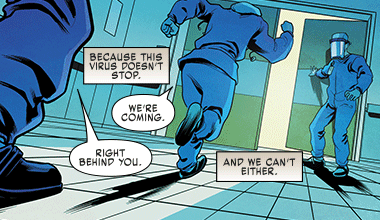This scene is a section from a comic book, depicting an intense moment inside a building, likely a hospital, rendered with a blue color theme. The panel captures three characters in blue uniforms and protective gear, including face shields. They appear to be healthcare workers, running through a pair of light-colored double doors shaded in blue. One character holds the door open as the others rush towards it. The scene is dramatized with a Dutch angle, adding to the sense of urgency. Text boxes placed strategically in the panel convey their dialogue: one character says, "Because this virus doesn't stop," another adds, "We're coming," and a third, partially out of frame, says, "Right behind you." Additionally, a text box reads, "And we can't either," emphasizing their relentless determination.